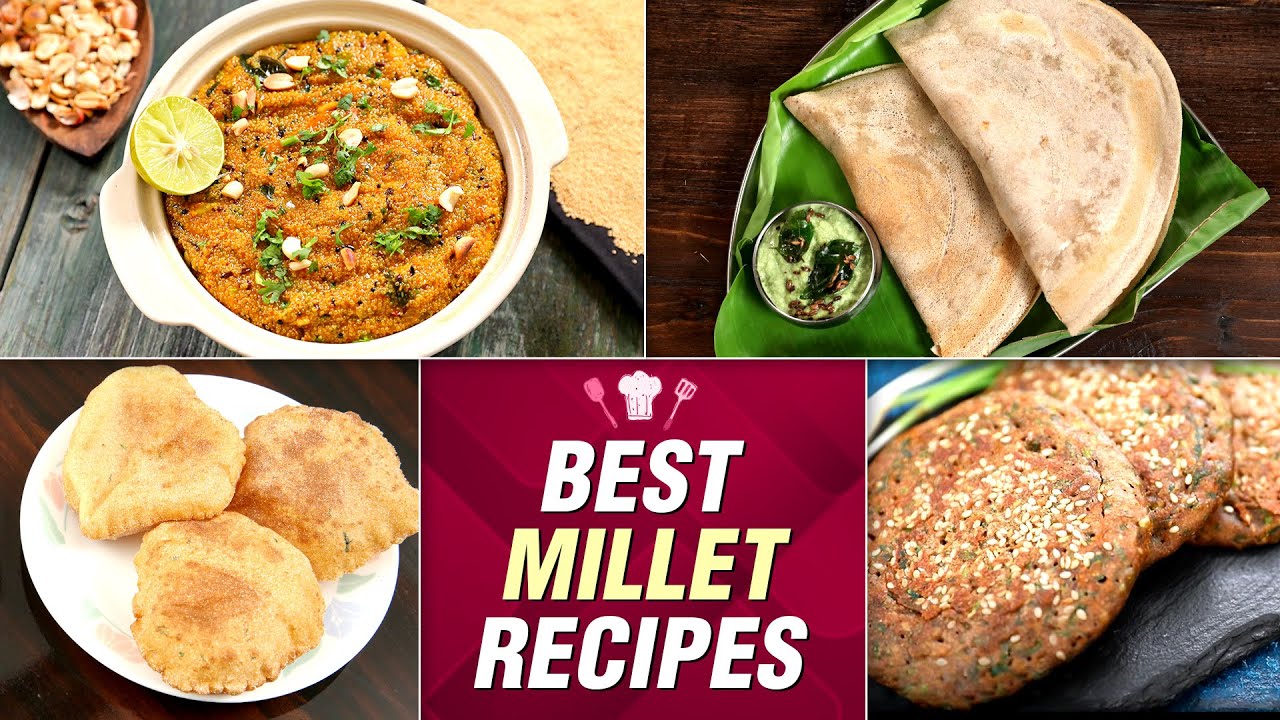This digital photograph displays a collage of four diverse millet-based dishes, framed under the text "Best Millet Recipes" in white font on a red background. In the upper left, there's a millet dish garnished with green vegetables, scattered small peanuts, a scoop, a lime wedge, and a baked good in a bowl. The upper right features millet wrapped in taco-like half circles on a green cloth atop a brown table. The bottom left image shows fried dough resembling croissants on a white circular plate. Lastly, the bottom right displays small, seeded millet cakes or patties. The overall color palette includes shades of brown, green, orange, red, white, and tan, bringing an appetizing and vibrant feel to the collection.